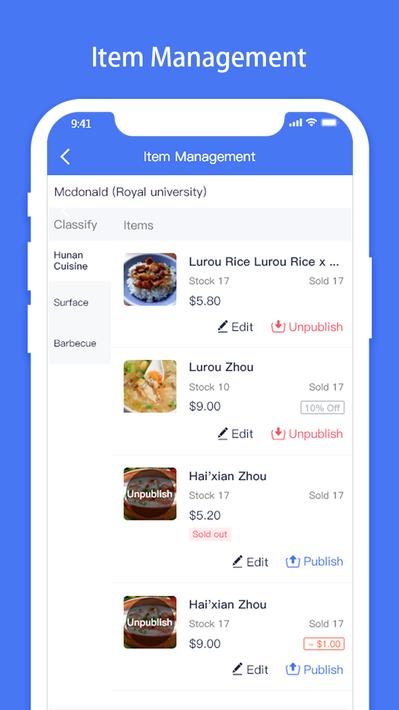The image is a detailed screenshot of a white smartphone with a blue background. At the top, the screen displays "Item Management" in white text, repeated in blue lettering beneath with a back menu button. The status bar indicates it is 9:41 AM, with full cellular signal, Wi-Fi, and battery levels. The phone is located at "McDonald's at Royal University."

The screen is showcasing an inventory management app with items categorized into "Hunan Can Cuisine," "Surface," and "Barbecue." Notable elements on the phone include three buttons on the left and one on the right side.

Below the categories, the screen lists the following items:

1. **Luau Rice**
   - SKU: LuauRiceX
   - Stock: 17 units
   - Price: $5.80
   - Units Sold: 17
   - Buttons: Edit, Unpublish

2. **Luau Rice**
   - SKU: LuauRiceX
   - Stock: 10 units
   - Price: $9.00
   - Units Sold: 17
   - Discount: 10% off
   - Buttons: Edit, Unpublish

3. **Hanxiang Xiao**
   - SKU: HanxiangXiao
   - Stock: 17 units
   - Price: $5.20
   - Status: Sold Out (in red)
   - Buttons: Edit (with a pencil icon), Publish, Delete (trash can with an arrow)

4. **Zao Haitang Xiao**
   - SKU: ZaoHaitangXiao
   - Stock: 17 units
   - Price: $9.00
   - Units Sold: 17
   - Discount: $1 off (in orange)
   - Buttons: Edit, Unpublish

Each listing includes stock levels, pricing, units sold, and options to edit, publish/unpublish, and delete, providing a comprehensive view of current inventory statuses and actions available.